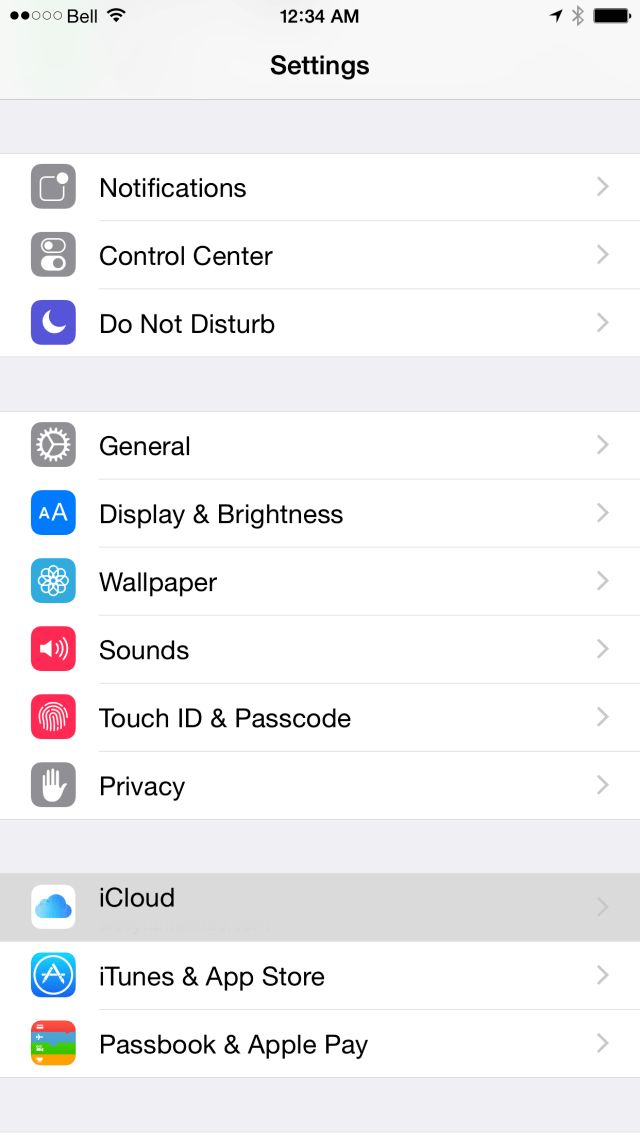The screenshot displays a smartphone screen captured at 2:34 AM, evidenced by the time indicator in the top center. The phone has a full battery, as shown by the battery icon in the top right corner, and a signal strength of two out of five dots in the top left. 

The screen is within the 'Settings' app, indicated by the word 'Settings' at the top. Below this, a thin gray separator bar divides the screen into sections. The first section features three options with icons to the left and right-facing arrows. These options are:
1. Notifications
2. Control Center
3. Do Not Disturb

Following another thicker gray bar, the second section displays six settings options with accompanying icons and right-facing arrows:
1. General
2. Display & Brightness
3. Wallpaper
4. Sounds
5. Touch ID & Passcode
6. Privacy

A lighter gray banner separates this section from the next. The third section highlights 'iCloud,' which is shown with a grayed-out appearance, indicating it is currently selected. Below this, two additional settings options, both with icons and right-facing arrows are listed:
1. iTunes & App Store
2. Passbook & Apple Pay

The bottom of the screen has a final gray blank area, rounding out the detailed view of the phone’s settings menu.